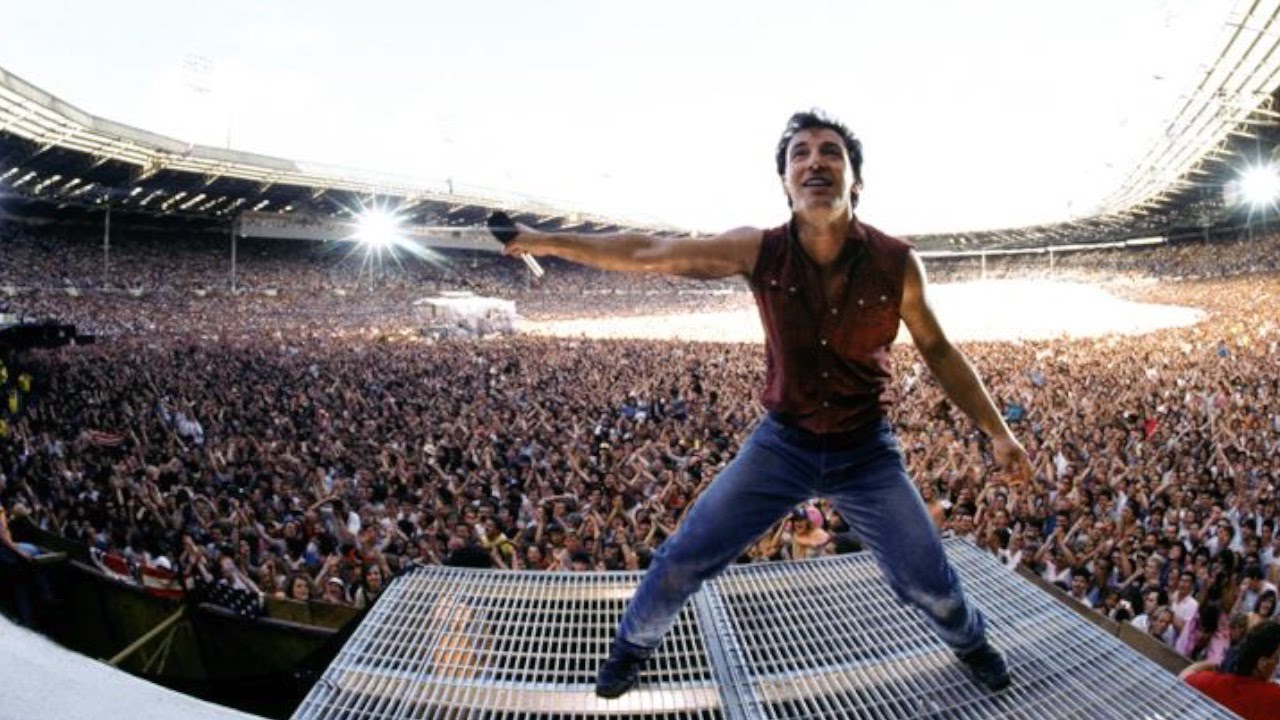In this dynamic fisheye photograph taken from the perspective of the stage, Bruce Springsteen, the iconic musician, is captured mid-performance in a packed open-air stadium. He stands prominently on a metal grid stage, situated on the right-hand side of the photo, facing towards the camera but looking to his upper right (our upper left). Springsteen is attired in denim blue jeans, black boots, and a sleeveless burgundy button-up shirt, which showcases his muscular build. His short, dark hair frames his face as he passionately extends a microphone in his outstretched right hand, engaging with the thousands of cheering fans surrounding him on all sides. Behind him, the expansive crowd fills both the ground and seating areas, creating a sea of excited concert-goers. The sky above is oversaturated, casting a dramatic white light over the scene, while two bright spotlights with starburst effects emerge from the bleachers. Additionally, an American flag is visible, draped over a security border wall on the bottom right of the photograph, adding a touch of patriotic flair to the electrifying atmosphere.